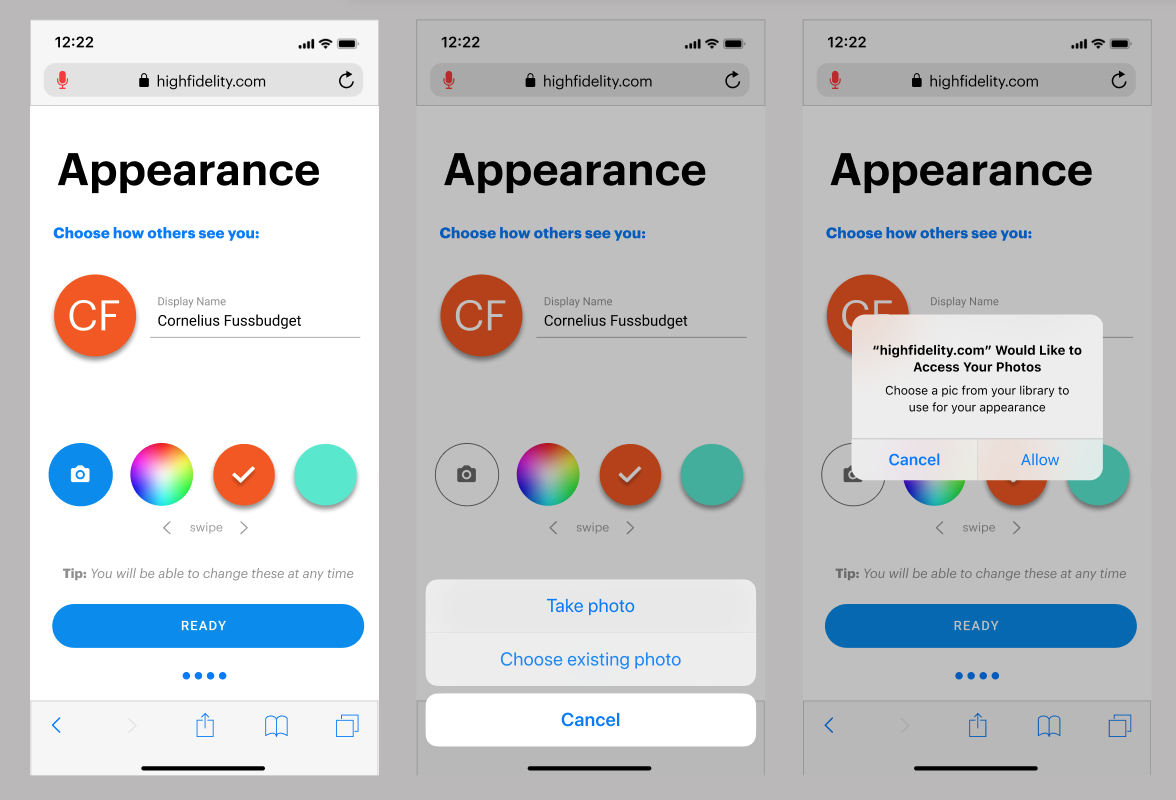In the image, there are three distinct sections arranged vertically, each featuring similar layouts and a few unique differences. The overall background for each section is gray, providing a uniform look.

In the top left corner of each section, the black time display reads "12:22," accompanied by black icons for the Wi-Fi signal, battery level, and reception signal. Below these icons, a gray rectangle is visible, housing a red microphone icon, followed by a black lock icon, and the text "highfidelity.com." Beneath this appears a marble crib image, topped by a thin gray line.

Centered within a white rectangular background, the black text "Appearance" is displayed, with a blue subtext underneath saying, "Choose how others will see you."

Each section contains a circle with differing contents:
1. **First Section:** The circle is blue.
2. **Second Section:** The circle is red with the white letters "CF."
3. **Third Section:** Similar to the second section, the circle is red with the white letters "CF."

Next to each circle is gray text stating "Display Name" followed by the name "Cornelius Budget" in black text.

At the bottom of each section:
1. **First Section:** Features a blue oval button labeled "Ready."
2. **Second Section:** Shows options in blue text: "Take Photo," "Choose Existing Photo," and "Cancel."
3. **Third Section:** Includes a blue oval button labeled "Ready" with an additional pop-up reading, "High Fidelity would like to access your photos. Choose a pic from your library to use for your appearance."

This detailed description captures the consistent layout and highlights the unique elements present in each of the three sections.